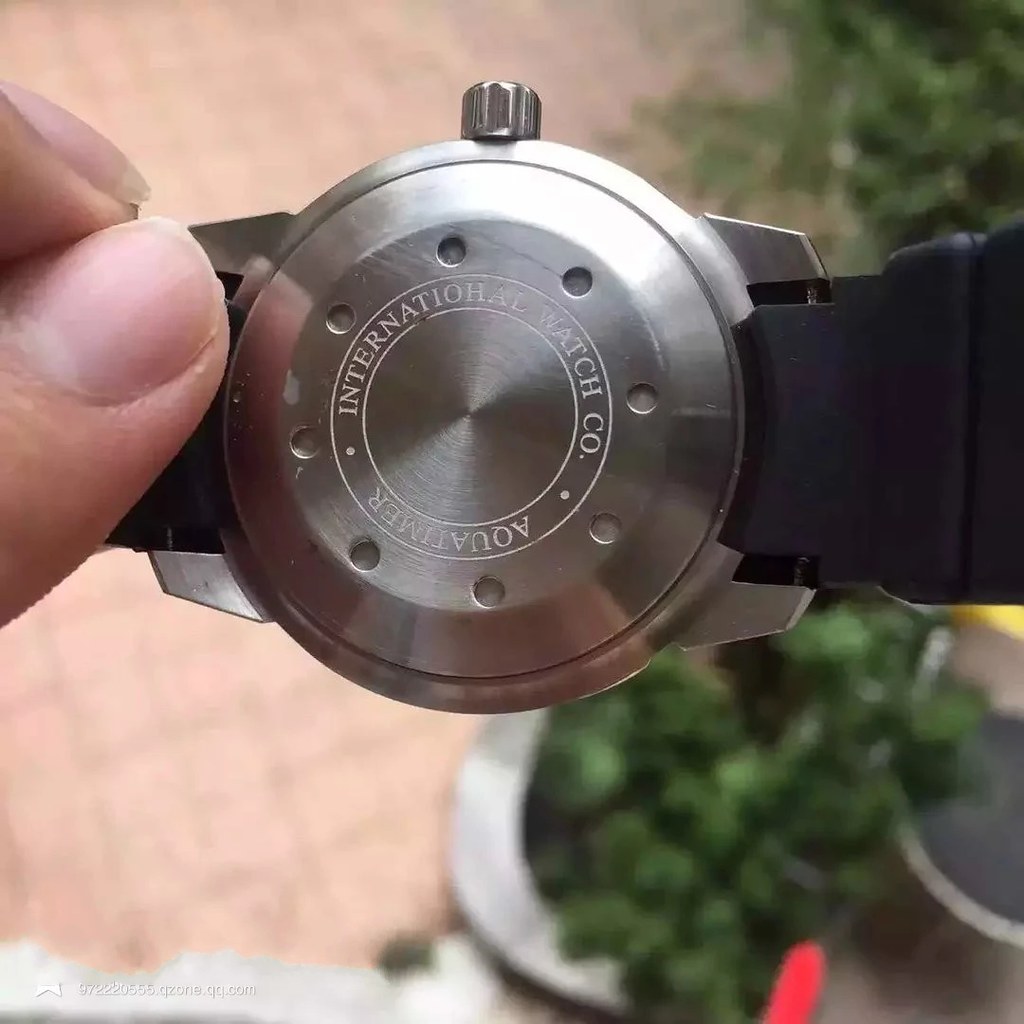The image depicts the back of a silver wristwatch with a black band, being held by a person whose pale thumb and forefinger are visible on the left side of the frame. The individual's nails are short and unpainted. The watch's band appears to be made of a rubber-like material. The watch's back features an engraved circular logo that reads "International Watch Co." with an additional upside-down inscription, "Aquatimer." The setting includes a background with a beige tiled surface, a small patch of grass, and several potted plants, including one in a white pot. Additionally, there is a blurred watermark in the bottom left corner, consisting of numbers and what appears to be an email address, "97222...@g-zone.qq.com."